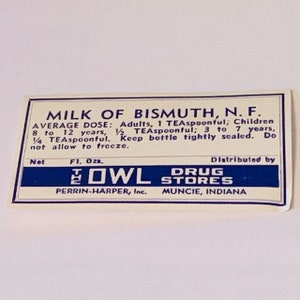The image depicts a vintage medication label, presumably from the 1950s or 1960s, set against a light grayish-blue background. The label, likely from a bottle, features a dark blue outline on a white background. At the top, bold dark blue letters read "Milk of Bismuth, N.F." Below this, detailed dosage instructions are provided: "Adults: 1 teaspoonful; Children 8 to 12 years: 1/2 teaspoonful; Children 3 to 7 years: 1/4 teaspoonful." Additional instructions caution to keep the bottle tightly sealed and to avoid freezing. Towards the bottom of the label, a dark blue banner with white text states "OWL Drugstores," followed by "Perry Harper Incorporated, Muncie, Indiana." This label includes information such as net fluid ounces and distribution details, reflecting its historical and utilitarian design.